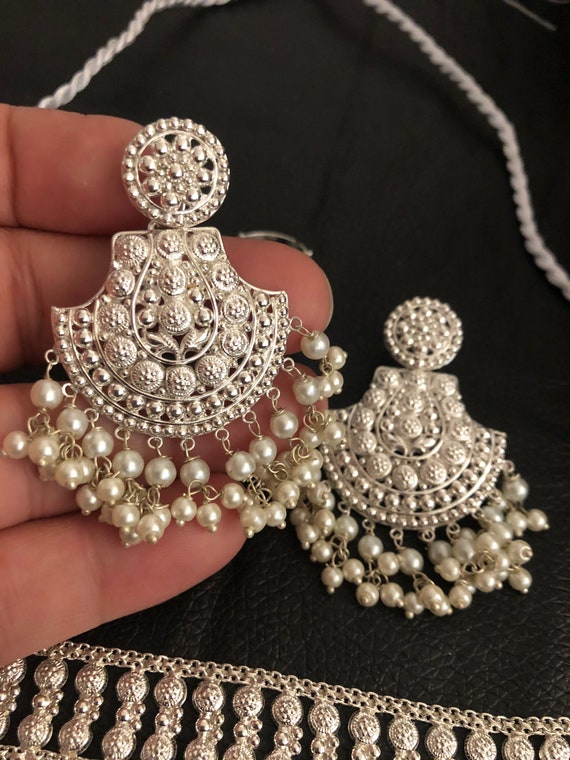In the image, a hand with four visible fingers extends from the left side, delicately holding a large, elaborate earring. The thumb is not visible. The earring features a round pendant at the top, transitioning into a fan-shaped, curved base adorned with intricate flowery designs. Small, white beads or pearls hang off the bottom in two rows. The background consists of a dark, ruffled material, likely fabric or leather. On the right side of the image lies an identical earring on the same dark material. Below the earrings, a gold chain with round pendant shapes stretches from left to right, and a white braided cord runs behind the fingers and loops downwards. This setup likely forms part of a matching jewelry set.